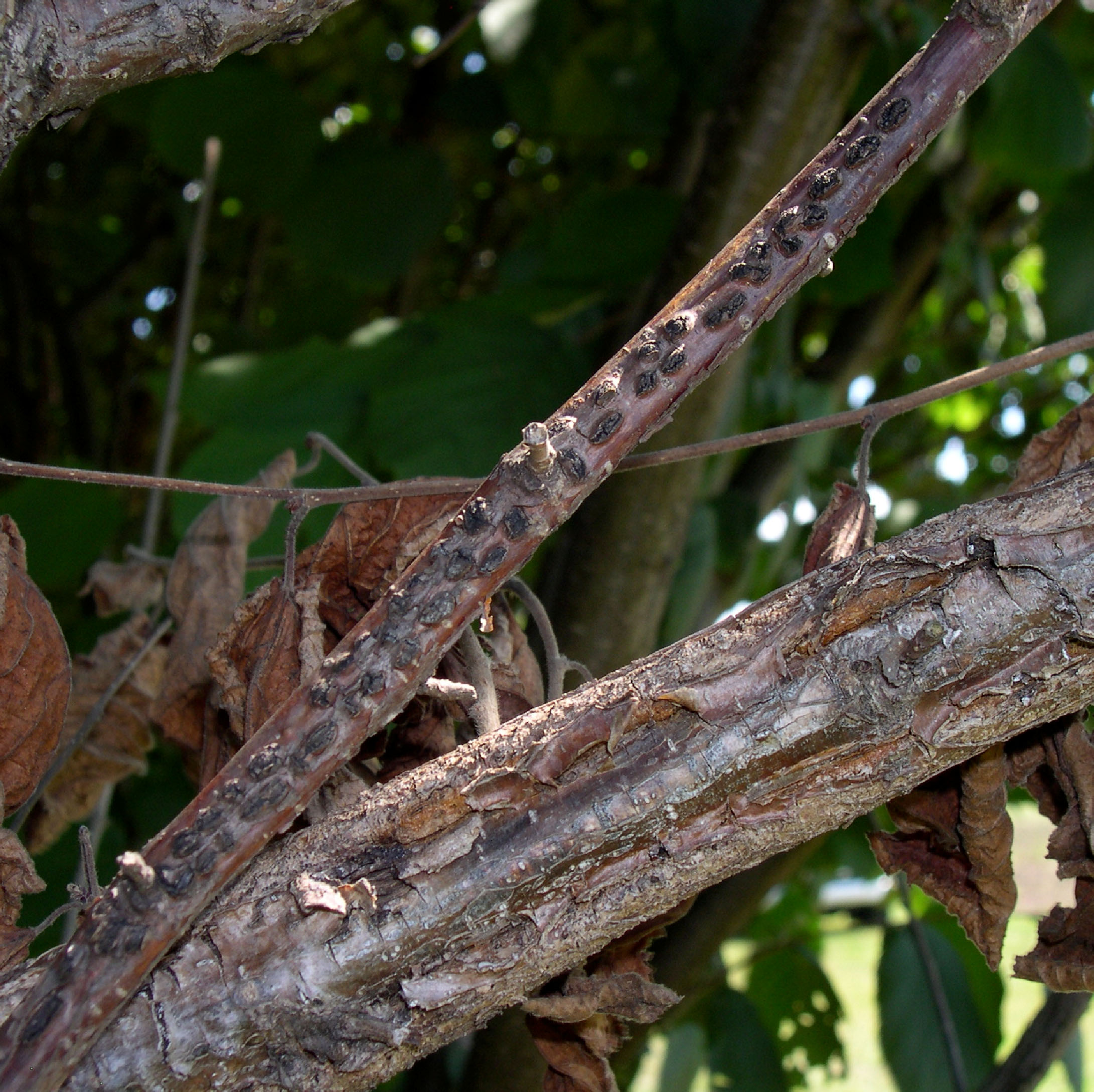The photograph captures a detailed scene of a tree with an intricate composition of branches and leaves. The background is filled with lush, out-of-focus green leaves, allowing patches of daylight to shimmer through. Dominating the foreground is a thicker, aged branch that leans to the right. This brown branch has distinctive white spots, suggesting possible bark peeling or some form of natural markings. Adjacent to it is a thinner, darker brown branch with curious black spots, adding to the textured complexity of the scene.

Further into the composition, a very thin branch with lifeless brown leaves indicates the inevitability of seasonal change or the aging of the tree. Additionally, a portion of another brown branch is visible in the upper left corner, enhancing the sense of depth. Towards the middle left portion of the picture, wrinkled orange leaves add a hint of autumnal decay. The middle lower section of the photograph reveals a stick with peculiar circular or oval shapes embedded in it, potentially markings or unique natural features that intrigue the viewer.

Overall, the image encapsulates a serene yet intricate view of nature's cycles, with the interplay of decay and life enveloped in a tapestry of green and brown hues.